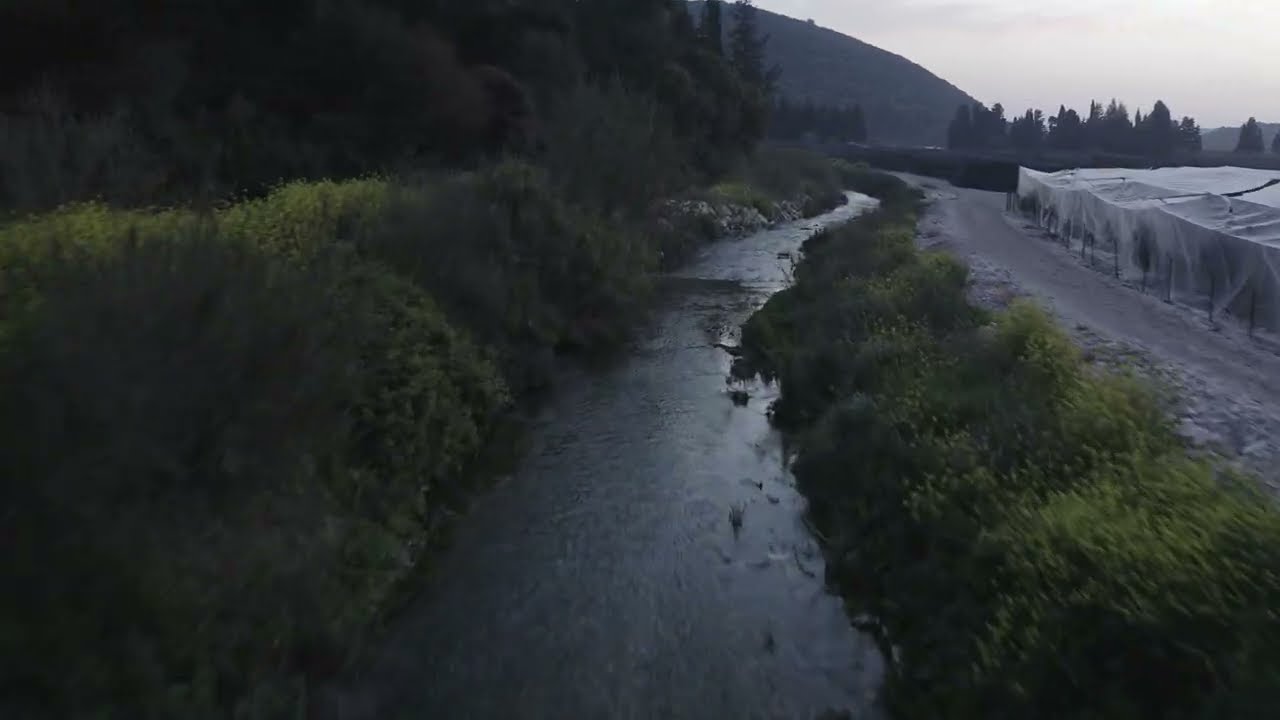The photograph captures a scenic view where a narrow, dark water stream flows through the center, flanked by dense greenery and trees. On both sides of the stream, the ground is adorned with lush plants, some of which bloom with vibrant yellow flowers. To the right of the stream lies a road, beyond which a building structure covered with transparent plastic can be seen. This structure resembles a tent and appears to be at the edge of the road, suggesting it might not be in regular use. Beyond the building, a tall forest of trees rises, creating a backdrop of rich green hues. In the distance, a hill emerges, under a sky that is white with scattered clouds. The overall image is brightly lit by daylight, accentuating the different shades of green in the foliage and the light gray-blue reflections on the water.